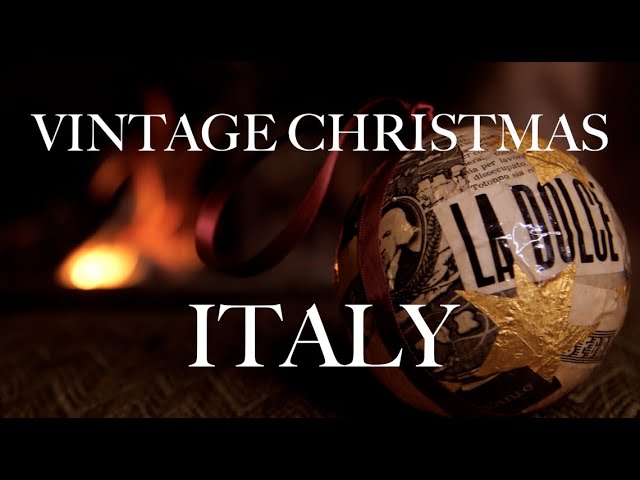This image, reminiscent of a vintage postcard, features the phrase "VINTAGE CHRISTMAS" in white uppercase letters across the top and "ITALY" at the bottom, both situated within a horizontal rectangular frame. Central to the photograph is a golden foil-covered Christmas tree ornament adorned with the words "LA DOLCE" in large black uppercase font on a white rectangular label. To the left of this ornament, captured within a small circular frame, is the image of an older gentleman with a powdered wig reminiscent of the 18th century. The background is predominantly dark and blurry, with a notable reflection of a flame or fireplace to the left, adding a warm, festive glow. The overall scene evokes a charming vintage Christmas ambiance, rich in dark, warm tones and a variety of colors including white, black, dark red, gold, blue, orange, and yellow.